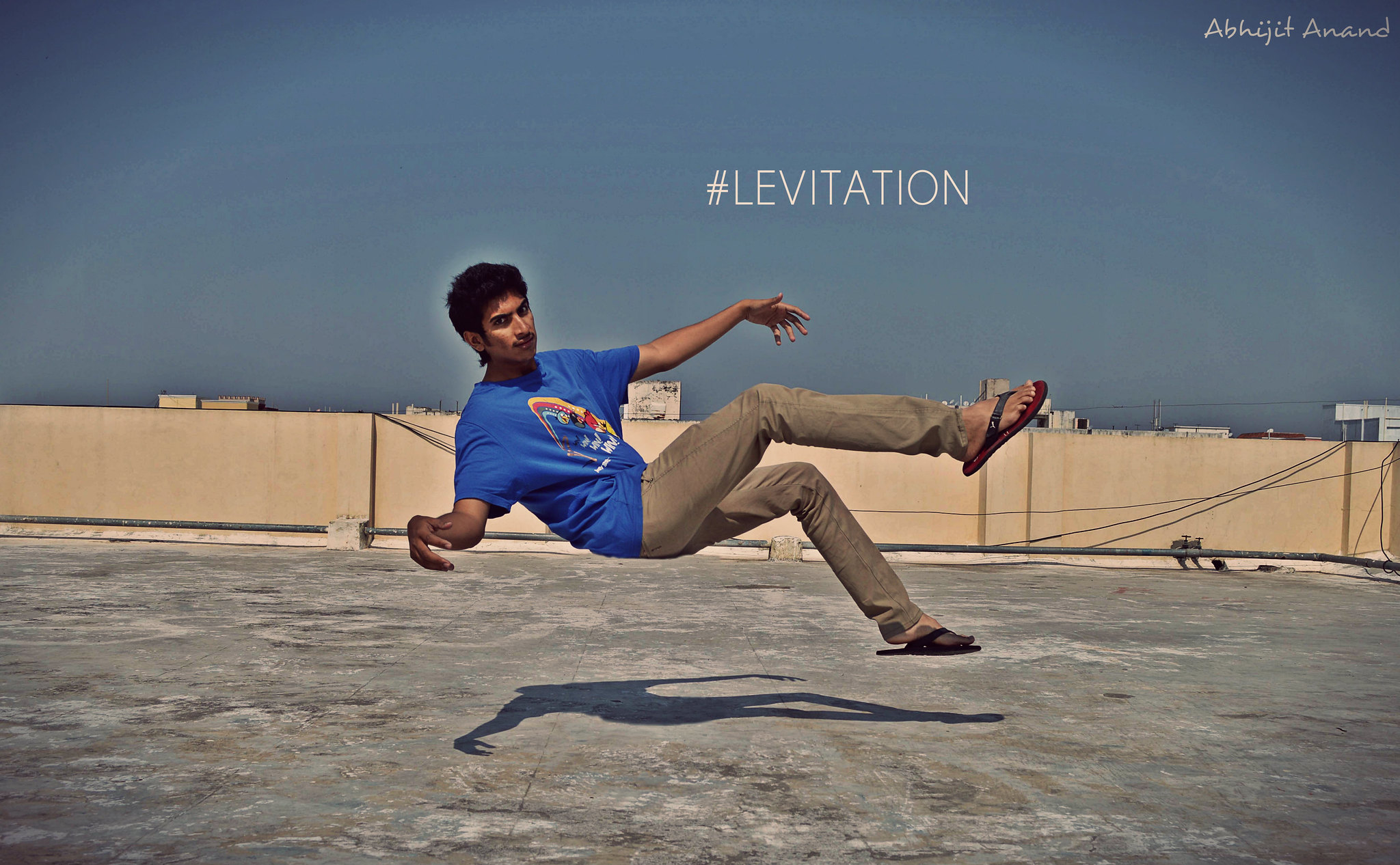The color photograph captures a man on the rooftop of a building, balancing on one leg with his other foot and both arms raised, creating an illusion of levitation. He wears flip-flops, khaki pants, and a blue short-sleeved t-shirt featuring a colorful design, while his dark hair and mustache are clearly visible. The man is positioned centrally in the image, with the background showing a tan wall of the roof, the tops of surrounding buildings, power lines, and a sunny sky taking up half the frame. Overlaying the man is a white hashtag reading "LEVITATION," and in the upper right corner, the photograph is signed by Abjit Anand in white lettering. The ground surface of the roof appears to be concrete, and the scene is set outdoors in the middle of the day, emphasizing the various shades of blue, white, tan, brown, red, orange, and gray present in the image.